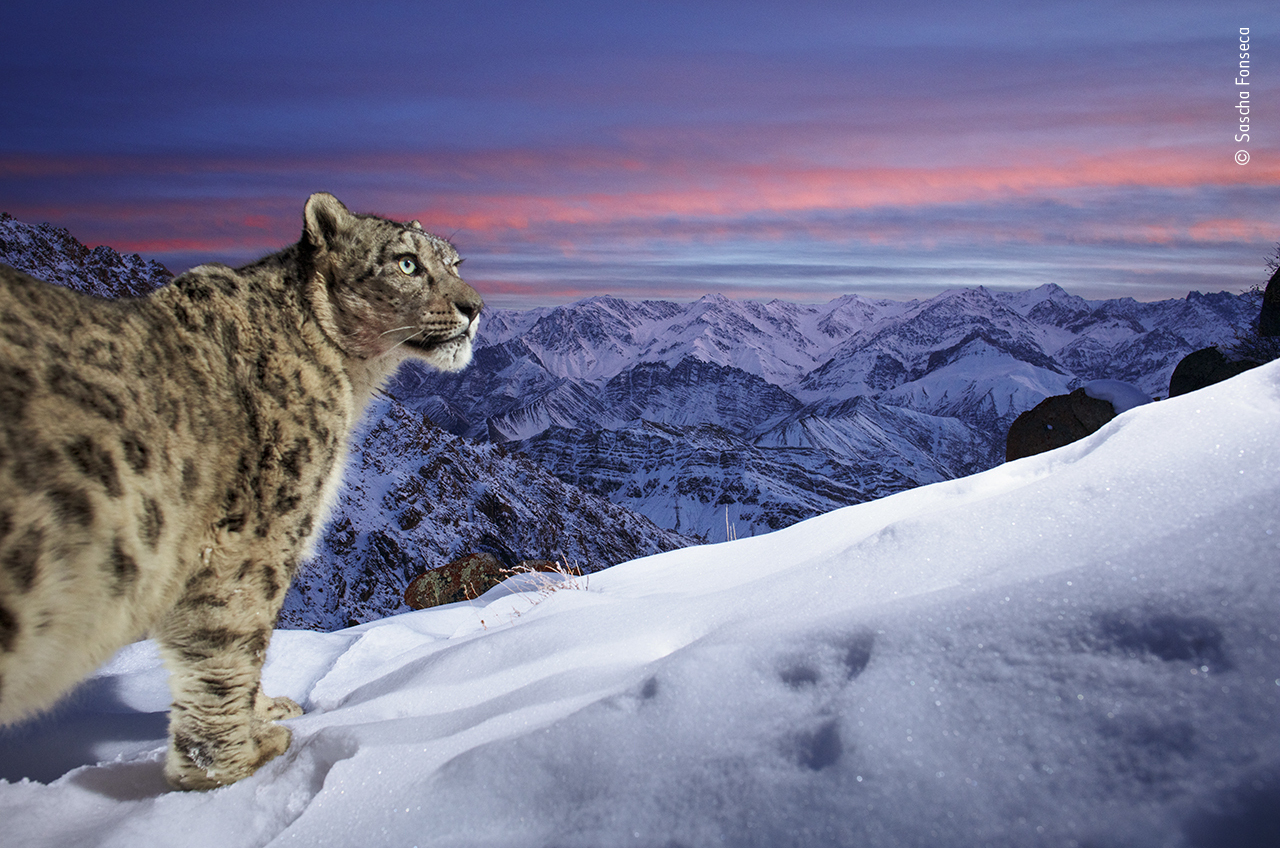The image captures a majestic snow leopard positioned on the left side, gracefully walking on a snowy mountain slope. The snow leopard's piercing light green eyes and black nose are beautifully highlighted, standing out against the pristine snowy backdrop. The animal is facing right, revealing a side profile that includes its head, upper body, and one of its front legs, emphasizing its powerful yet elegant physique. The snow around the leopard sparkles, reflecting the soft light. In the background stretches a breathtaking vista of snow-capped mountains, dotted with trees on the right, and a prominent brownish-golden rock just behind the leopard. The sky above transitions between shades of blue and reddish-pink, indicating a serene sunset or sunrise. Pink clouds scattered across a blue sky add a dreamy quality to the scene, completing this stunningly detailed and tranquil wilderness portrait.